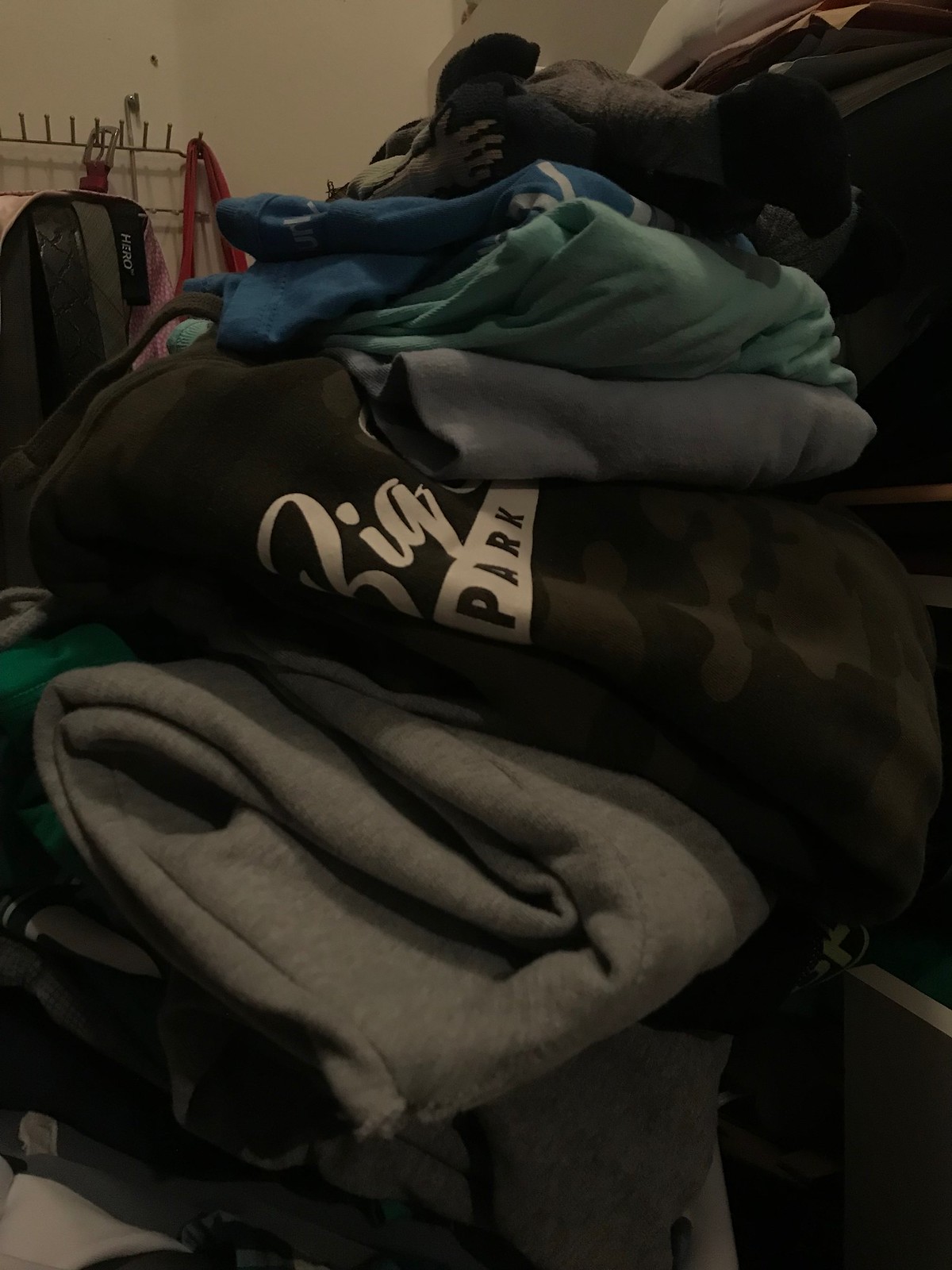This image depicts a mixed pile of folded clothing, predominantly featuring sweatshirts and athletic wear. Highlighted in the foreground is a gray sweatshirt, topped with a black sweatshirt that bears the word "PARK" in bold black letters within a white banner. Further up the stack, there are various other garments, including teal, blue, and black pieces, some of which are made of jersey material. A camouflage-patterned top is also visible, adding to the diverse collection of colors such as green and turquoise. The background showcases a white wall with part of a metal rack on the left, from which a red strap, a belt buckle, a pink tote bag, and a backpack hang, contributing to the cluttered yet casual setting. This assortment of clothing, potentially being organized for a giveaway, presents a vivid snapshot of everyday wear and storage.